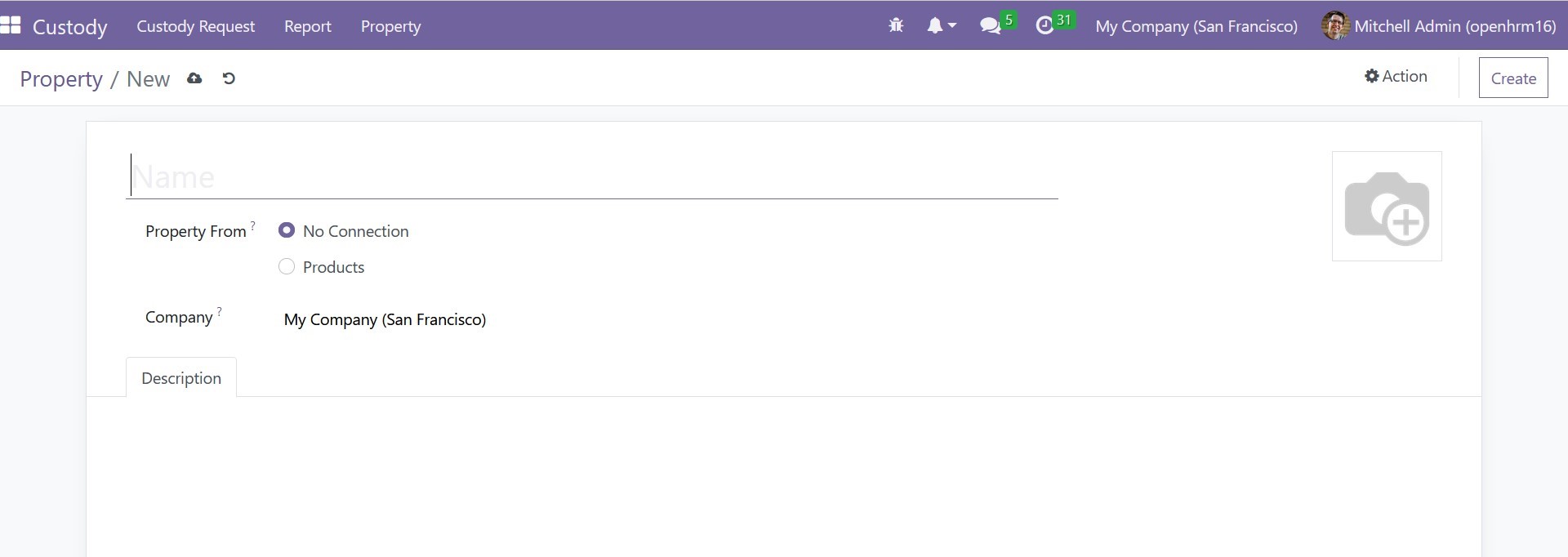The image features a horizontal, rectangular header in a medium-tone purple background that spans from left to right at the top. On the upper left-hand side, there is a white logo followed by the word "Custody" in white font. Adjacent to it are the terms "Custody Request," "Report," and "Property," all in white font. Moving right of center, a series of icons appears, all in white, with the last two icons having small green squares attached to them. Further to the right, it reads "My Company (San Francisco)" in white font. 

Adjacent to this text, there is a circular picture placeholder, followed by some text that is not fully legible. Below this header section, on a crisp white background, the text "Property / New" is displayed alongside an icon. On the right side, a Settings button appears, followed by the terms "Action" and "Create," with "Create" being highlighted in a white box outlined in dark coloring.

The main section of the page features a clean white area set against an off-white background. A light gray horizontal line runs across the top, accompanied by a single vertical line at the beginning. To the rightmost part of this gray line, there is a camera icon. Below the horizontal line, the text "Property From" is present, offering two choices: "No Connection" and "Products." The "No Connection" option is indicated with a colored circle leaving a white dot in the center. On the left side of this section, it reads "Company," while on the right, it reiterates "My Company (San Francisco)." Beneath this, there is a tab labeled "Description."